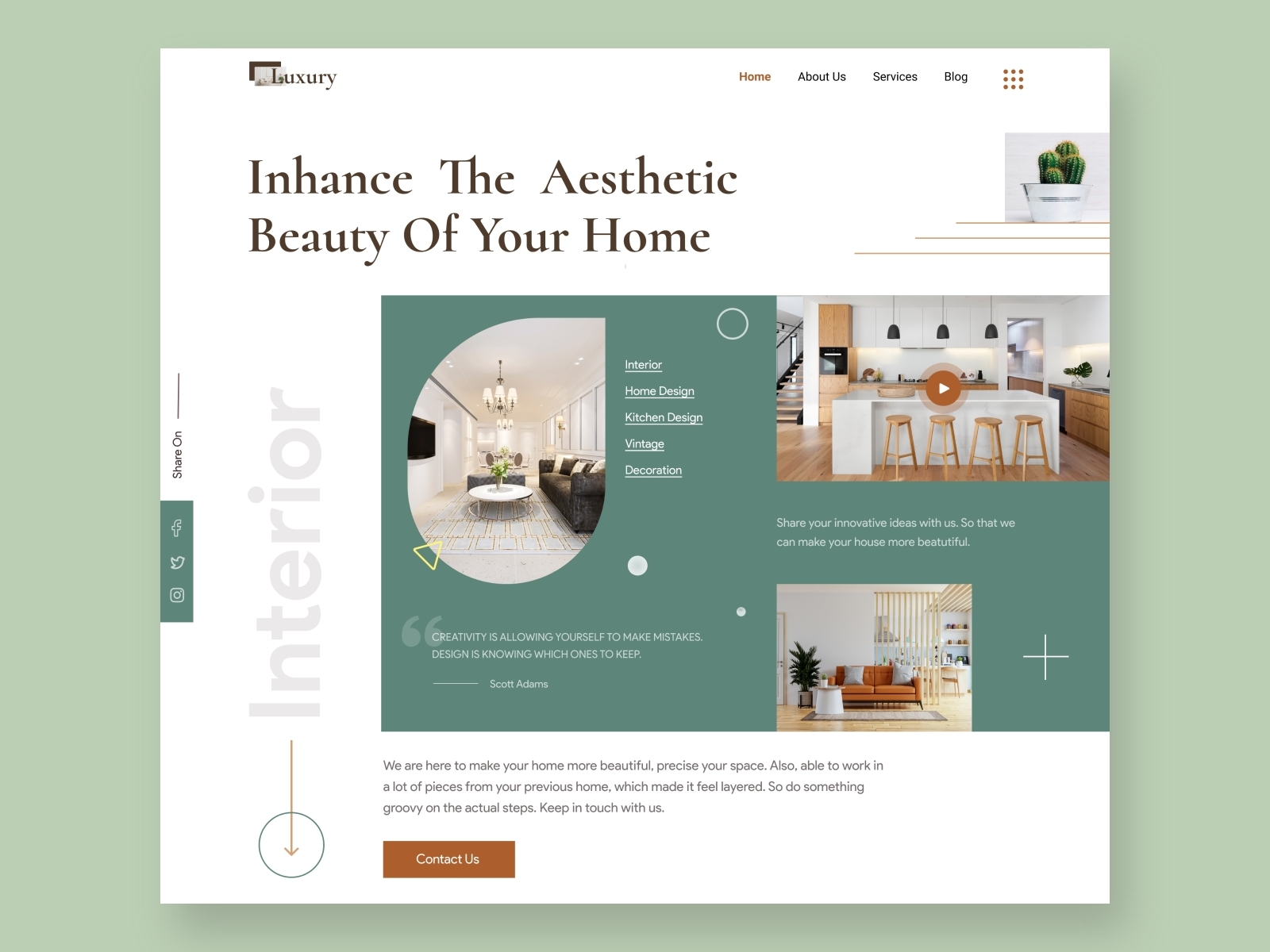The image features a website layout with a light green background and a border that is wider on the left and right sides compared to the top and bottom. The central portion of the layout is framed by a white background. At the top right corner, there are navigation options: "Home," "About Us," "Surfaces," and "Blog." The "Home" option is highlighted in brown, while the others are in black. A nine-dot icon in brown is also present in the top right corner.

In the upper left corner, the word "Luxury" is displayed. Below it, in brown text on a white background, is the tagline "Enhance the Aesthetic Beauty of Your Home." The word "Interior" appears in gray, oriented vertically down the left side.

A green section with white font features the following points: "Interior Home Design," "Kitchen Design," "Vintage," and "Decoration." A quote from Scott Adams reads, "Creativity is allowing yourself to make mistakes. Design is knowing which ones to keep." An invitation is extended to share innovation ideas to make homes more beautiful.

Below the text, there are images of various home interiors:
1. A kitchen with white cabinets and brown bar stools.
2. A living space with an orange sofa, two gray pillows, and an area rug.
3. A chic room featuring a brown sofa, a chandelier over a table, and a white and gold rug.

At the bottom, the text reads: "We are here to make your home more beautiful. Precise your space, also able to work in a lot of pieces from your personal home or previous home, which makes it feel layered. Do something groovy on the actual steps. Keep in touch with us." There is also a call to action with a "Contact Us" button.